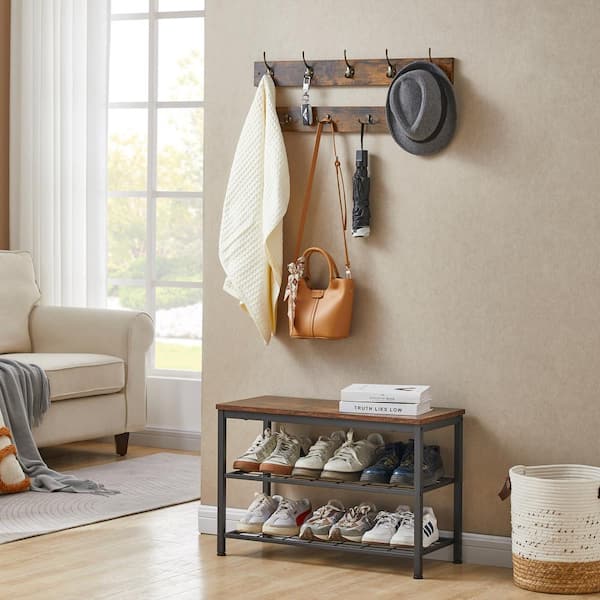The image depicts a cozy corner of a home interior, likely adjacent to a door, partially revealing a living room area. The focal wall features a mounted rack adorned with various items: a gray fedora on the far right, a small black umbrella to its left, a tan beige handbag with a long strap hanging further left, a keychain or keys above to the left of the handbag, and either a shawl or a jacket next to the keys. Below this rack is a shoe rack with metal legs and frame, dark gray with a wooden top. The rack houses six pairs of tennis shoes, three on each of the two shelves, and on top of it, there are two books, one possibly titled "Truth Lies Low." Also on top of the rack is a basket, potentially for wet items or umbrellas. To the left, partially visible, are a cream-colored sofa with a gray shawl or blanket draped over it, an area rug in front, and sheer white curtains hanging over a French pane-style window. Daylight streams in, revealing a tree outside, suggesting a serene and organized space inside.